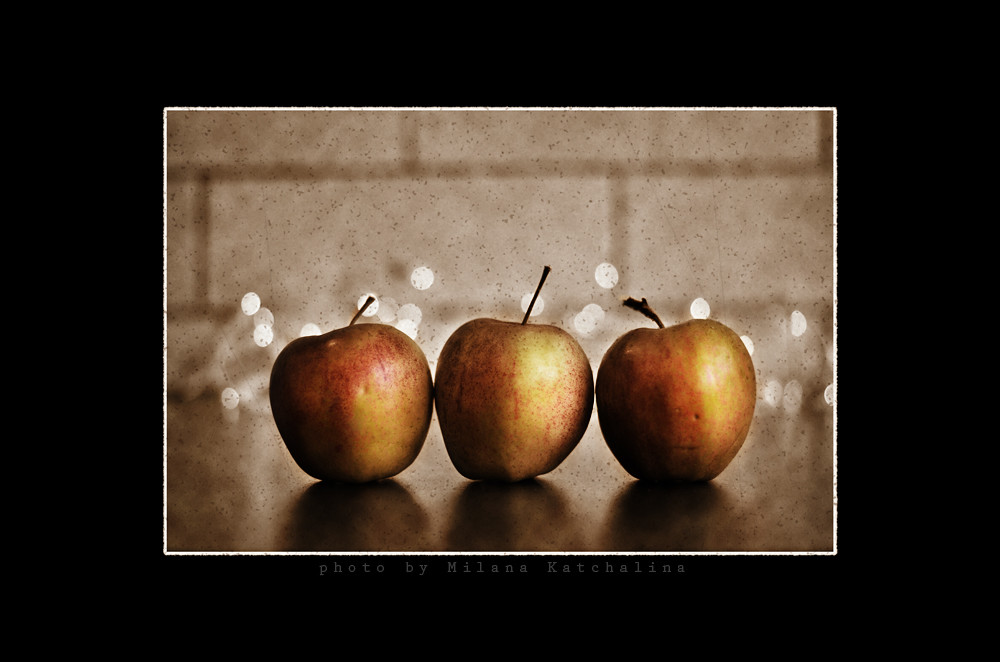This is a detailed photo of three apples, with distinct red and yellow hues, set side by side on a marble countertop. The apple in the middle has a noticeably larger stem. In the background, there's an off-white brick wall adorned with subtle black dots, adding a textured dimension. Sparkling glassware catches the light and glimmers against this backdrop, while white, illuminated Christmas lights or tinsel add a festive touch. Framing this visually rich scene is a thin white border, and a small gray caption at the bottom identifies the photographer as Milana Kata Chalina.